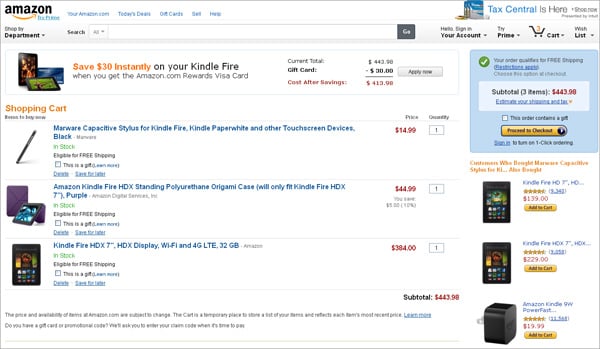The image depicts an Amazon webpage, characterized by the prominent Amazon logo in big black letters in the upper left corner, accompanied by the iconic golden arrow that points from left to right. At the top right corner, there are small blue clickable categories advertised under the label "tax central is here." Below this, a promotional banner in orange highlights a $30 savings offer on a Kindle Fire when you obtain the Amazon.com Rewards Visa Card, showing detailed calculations of the potential savings.

A shopping cart summary reveals three computer-related products. The first item is a black desk stylus priced at $14.99. The second item listed is an Amazon Kindle Fire, costing $44.99. The final item is a more expensive Kindle Fire with Wi-Fi, priced at nearly $400, bringing the total amount to $443.99.

On the right side of the webpage, additional images suggest other items available for purchase on Amazon.